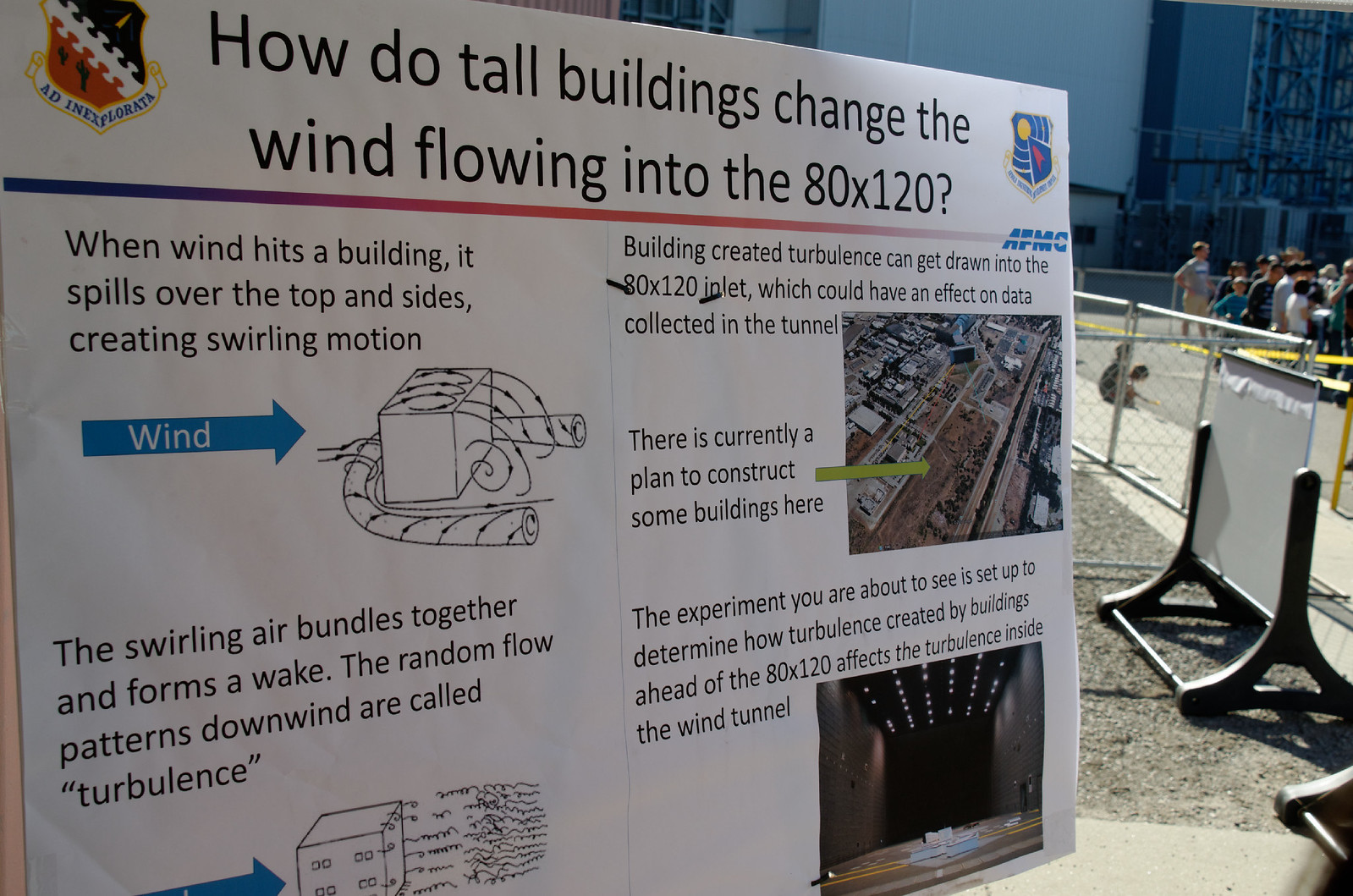In this image, a white billboard sign with black text prominently asks, "How do tall buildings change the wind flowing into the 80 by 120?" The sign is positioned on the left side of the picture and contains detailed explanations about wind behavior around tall buildings. The text and accompanying diagrams illustrate how wind hits a building, spilling over the top and sides to create a swirling motion. One diagram, highlighted with a blue arrow labeled "wind," depicts this swirling effect. The sign further explains that these swirling air currents bundle together to form a wake, leading to random flow patterns known as turbulence. This turbulence, generated near the structures, can be drawn into the 80 by 120 inlet, potentially affecting data collected in the associated wind tunnel experiment. The bottom of the sign mentions a plan to construct buildings in the area and notes the purpose of the experiment, which is to determine how such turbulence impacts the tunnel.

To the right side of the picture, a group of people is standing in line, likely awaiting entry into the site. The area is secured with a fence and division tape, hinting at ongoing construction. These contextual details add to the narrative of an active, controlled experimental environment where the effects of newly constructed buildings on wind patterns are being studied.